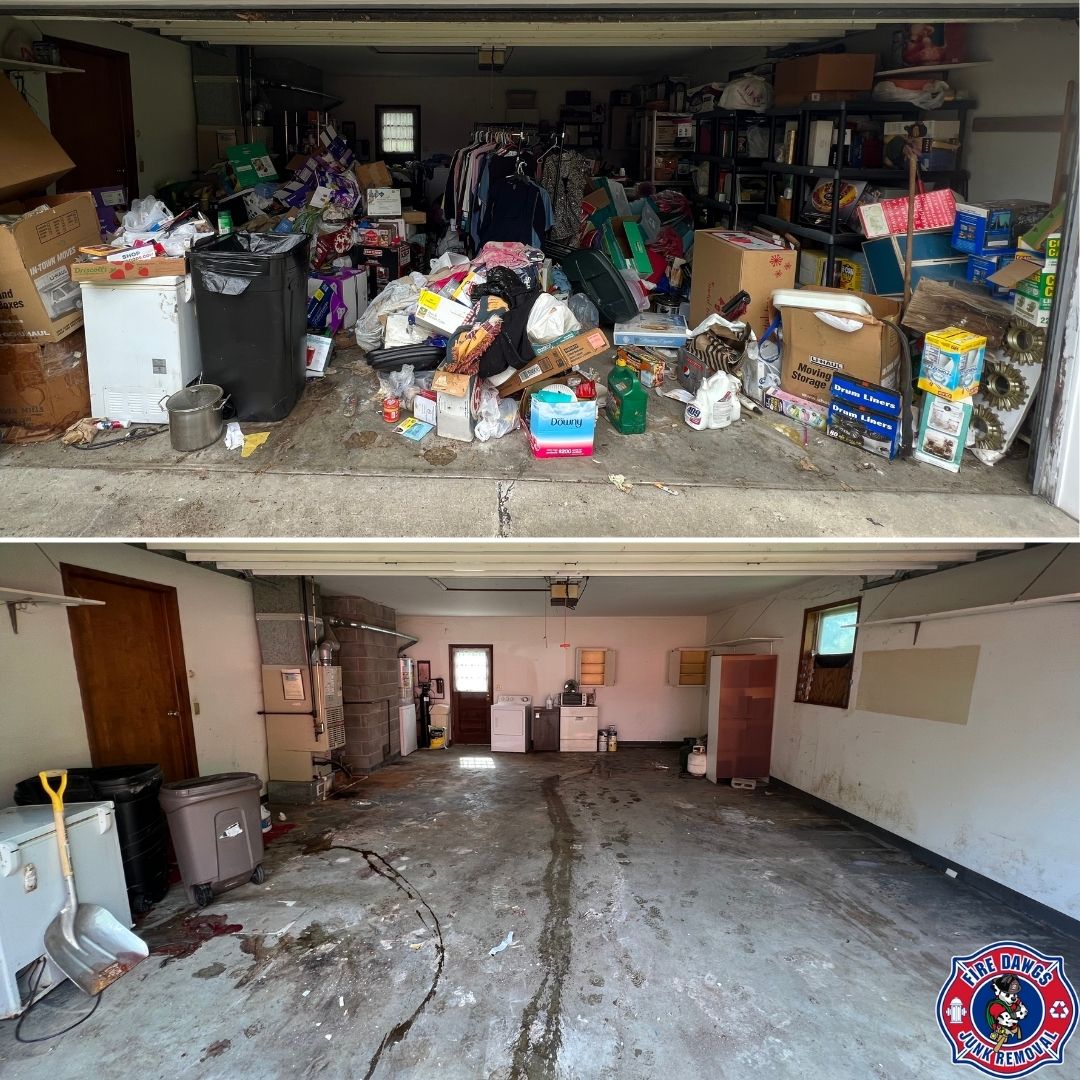The image is a comparative before-and-after set of photographs depicting a transformation of a cluttered garage into an organized and clean space. In the top photograph, the garage is packed with various items including boxes, shelving units, trash bins, holiday decorations, clothing racks, plastic bags, and metal pots and pans. The clutter obscures much of the garage interior, but you can spot a light-colored concrete floor and brown wooden doors on the left side and at the back. The garage door is open, revealing the overwhelming amount of stuff inside. 

In the bottom photograph, the same garage has been entirely cleaned out. The clutter is gone, leaving the floor and walls visible. Essential items like a garbage can, a snow shovel, and an old refrigerator remain on the left side, and the washer and dryer are now clearly visible at the back. The shelves are empty, the space is open, and more light shines through. The lower right corner of this image displays a logo resembling a firefighter emblem with a Dalmatian, and it reads "Fire Dogs Junk Removal," indicating that a junk removal service facilitated this impressive clean-up.